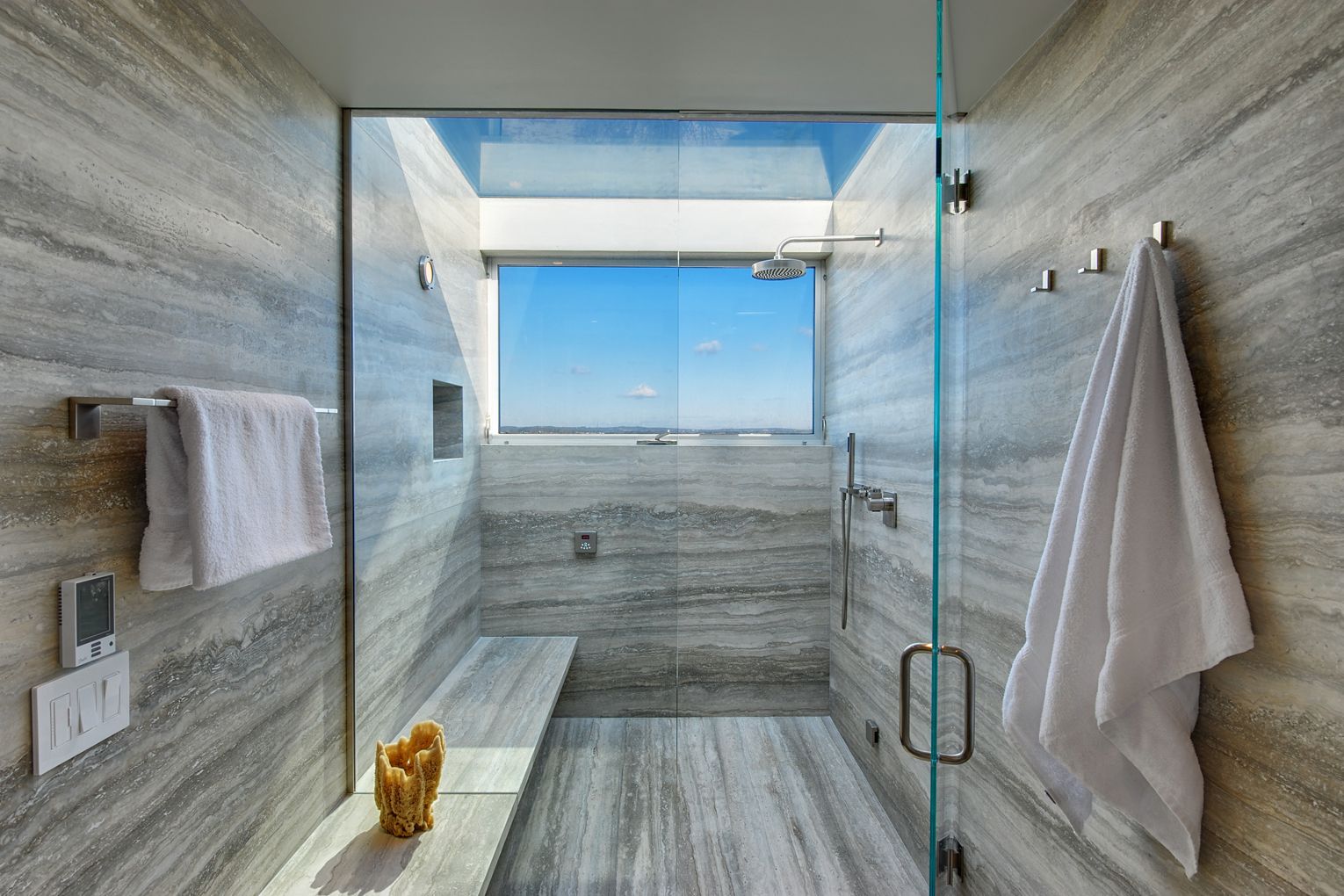This is a photograph of a luxurious, custom-built, walk-in shower that exudes modern elegance. The shower features a combination of materials that give it a sophisticated appearance, with walls crafted from ceramic tiles designed to mimic light to darker brown wooden planks, displaying a straight-lined pattern. The spacious shower is enclosed by a sleek, thin glass door with a handle, providing an unobstructed view. On the right-hand wall, there are three hooks, with one towel hanging on one of them. To the left, a towel rack holds another towel, located just above three light fixtures. 

A rather large glass window at one end of the shower allows an impressive view of the blue sky with clouds, introducing ample natural light. Additionally, the top of the shower features a skylight that maximizes the airy open feel, though it may permit visibility into the shower from above.

Inside the shower, there is a luxurious marble-like bench and sleek, minimalistic features, including a showerhead and an additional sprayer. The shower wall includes a recessed niche for storing soaps and shampoos, though it appears currently empty, contributing to the shower’s extremely sparse and clean look. Complementing the modern amenities is a small candle placed on a bench outside of the shower, adding a touch of warmth. The design is accentuated further by the strategic positioning of towels, lighting, and what might be noted as a thermostat on the left side, ensuring both function and style in this contemporary bathing space.